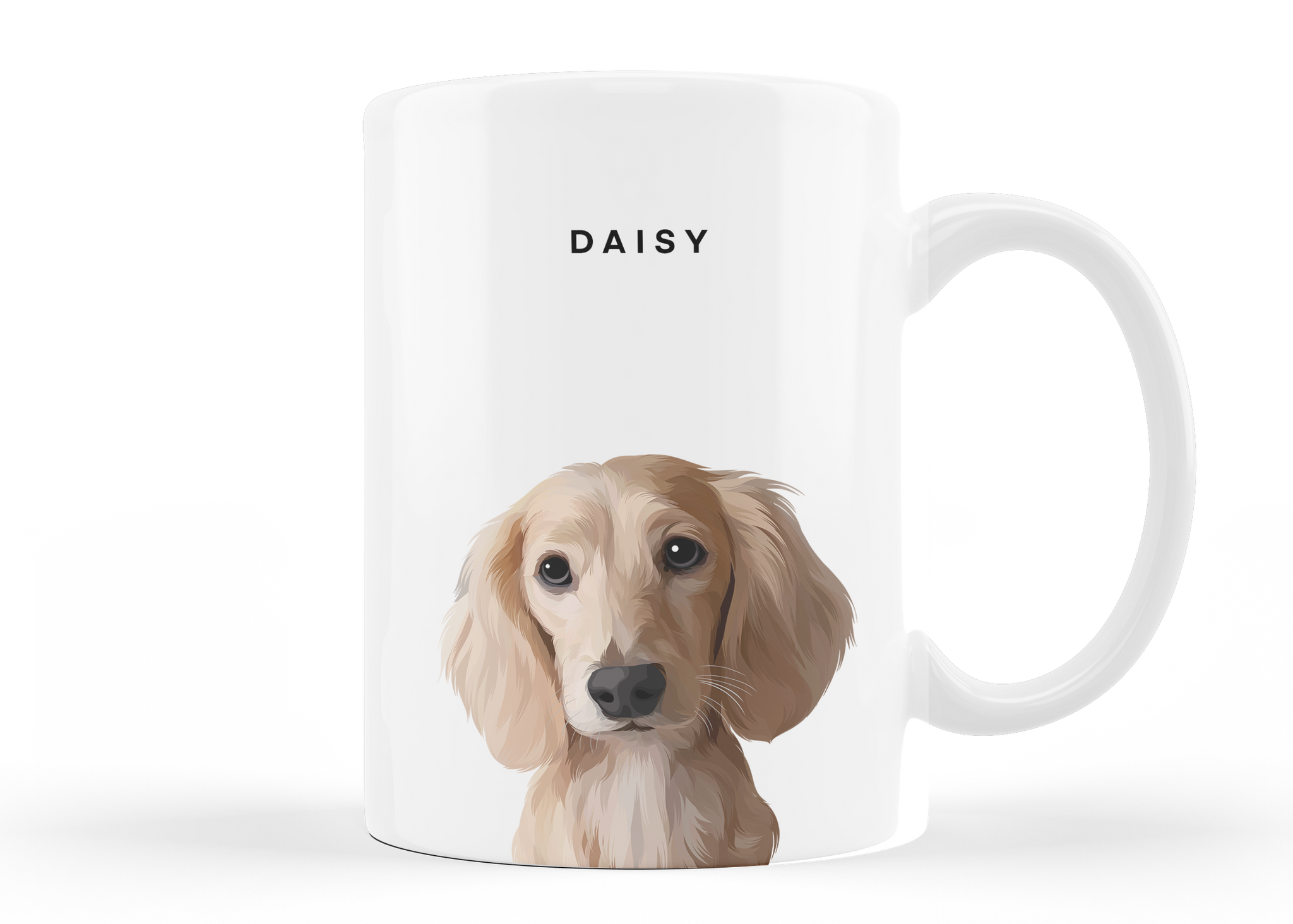This photograph features a white, porcelain coffee mug against a similarly white background, with its handle positioned on the right side. Centered on the mug, in bold black lettering, is the name "DAISY". Below the text, there is an impressionistic digital art rendering of a golden retriever or Labrador puppy, looking directly ahead. The dog, with its slightly smudged watercolor-like appearance, has fluffy, drooping ears, and a distinctive flat head with a pronounced snout. The coloring of the dog varies between shades of gold, beige, and white, with contrasting black eyes, nose, and subtle mouth details. The artistic depiction likely draws from a real photograph, embracing a semi-realistic style that captures the essence of a playful, yet slightly matured puppy. The mug is lit from multiple angles, creating soft shadows on either side, enhancing its shiny exterior.